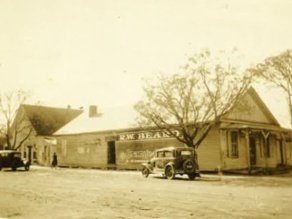This sepia-toned, digitally-preserved photograph, likely from the early 1900s, captures a detailed scene of a family-owned general store. The original high-quality photo features a large, one-story log cabin-like building with an angled roof, bearing the sign "R.W. Beard" painted on its side near a door. The image shows two old cars, presumably from the 1910s or 1920s, parked or driving by on a dirt road in front of the store. The surrounding landscape includes a couple of trees, although they appear without leaves, adding to the vintage ambiance of the image. A single individual dressed in dark clothing stands on the left side of the photo, enhancing the historical context. The residential home connected to the store suggests it was a self-sustained business where the owners lived and worked. The sky is a light off-white, indicative of the oxidation process affecting old black-and-white photos, and there is a mix of white and dark patches on the roof, further emphasizing the photograph's age.